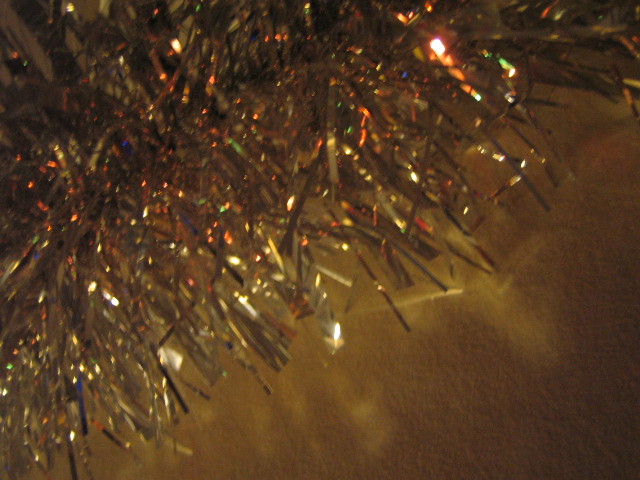This photograph is a zoomed-in view of a poorly lit and low-quality Christmas tree, adorned with silver tinsel and colored lights. The image predominantly showcases the green needles of a pine tree, which fill the top left, bottom left, top right, and center of the frame. The lower right corner of the image is notably dark and blurry, fading from black to a brownish-gold and finally to a lighter yellow hue as it approaches the tree. The tinsel catches the light, creating shimmering reflections that add minor splashes of orange, green, and blue against its silver surface. A single red Christmas light near the upper portion of the image enhances the tinsel's shine, contributing to its festive glow.